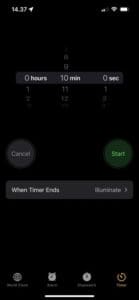This image captures a highly blurry screenshot of a timer application on a smartphone, set against a pure black background. The top left of the header, displayed in white, reads "1437" with an arrow pointing diagonally upwards to the right. On the top right of the header, you can identify a two-bar filled mobile data icon, a fully filled Wi-Fi icon, and a fully charged battery icon.

Occupying the top third of the frame is the time selection area, which is divided into three columns. The leftmost column indicates hours, starting at zero and fading down to one and two in a gradient into black. The middle column represents minutes, showing a highlighted '10' in the center, with numbers incrementing upwards from nine to eight and downwards from 11 to 12 and 13, also fading into black. The right column specifies seconds, abbreviated as "SEC," beginning at zero and gradually fading down from one to three.

A gray box highlights the selected time at zero hours, ten minutes, and zero seconds. Below this section are two circular buttons: a gray circle labeled "Cancel" on the left, and a green circle labeled "Start" on the right. Further down, a gray rectangle displays the text "When timer ends," with the word "Illuminate" slightly darkened to its right and accompanied by a rightward arrow.

The bottom of the screen, set against a black footer, features four icons, although their details are obscured by the blur.